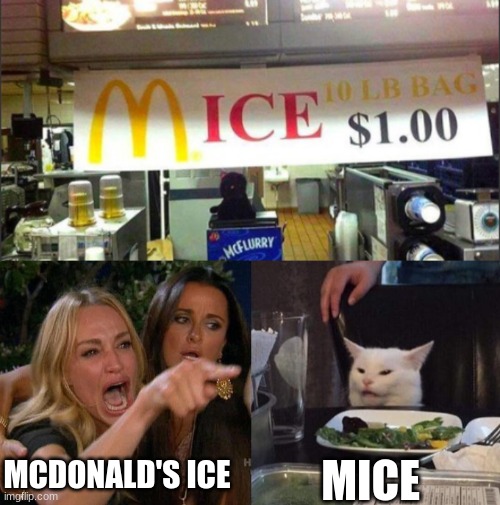The image meme consists of three segments: at the top, a professional-looking photograph depicts a McDonald's kitchen, complete with kitchen equipment and a McFlurry machine noticeably labeled with "McFlurry" in white text on a blue surface. Dominating this top portion is a McDonald's advertisement banner. The banner prominently features the McDonald's golden arches logo, alongside bold yellow text that reads "Ice, 10 pound bag for a dollar," though the placement of the text causes it to appear as "Mice."

Below this, the meme itself is laid out in two smaller photographs side by side. On the left, an image captures a hysterical woman being restrained by another woman, with white text above her exclaiming "McDonald's Ice." On the right, a comical image shows a cat looking at a plate of food with white text above it that reads "Mice," playing on the visual pun established in the top banner.

In essence, the meme humorously juxtaposes the professional McDonald's advertisement with the viral "woman yelling at a cat" meme to create a mix-up between "McDonald's Ice" and "mice."